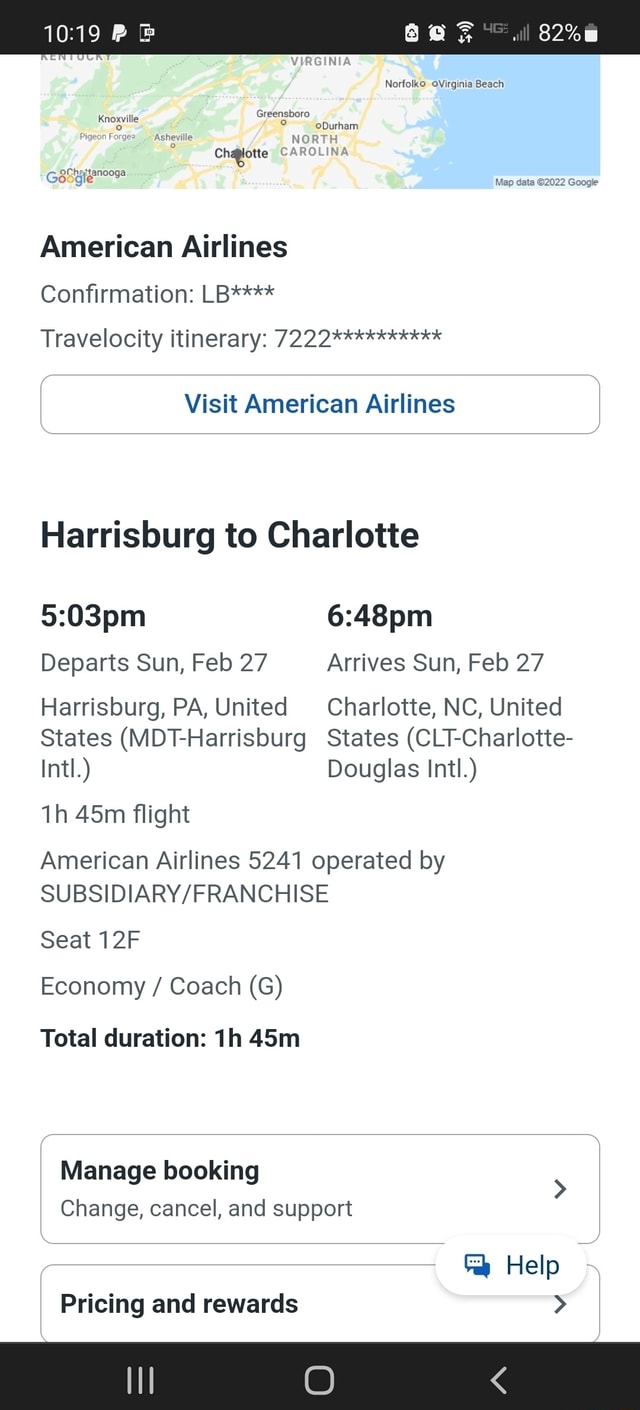A smartphone user's screenshot displays detailed travel information for an upcoming flight. The top edge of the screen shows a black status bar. On the left, it reads "1019," accompanied by a PayPal icon. On the right, various status icons are visible: a battery indicator, an alarm clock, a Wi-Fi signal, and a network coverage symbol.

Dominating the upper portion of the screenshot is a map featuring a pin near Charlotte, North Carolina. Below the map, the heading "American Airlines" is prominent, followed by a partially obscured confirmation code "LB****" and a Travelocity itinerary number "7222*****."

The main content provides detailed flight information:

- **Airline:** American Airlines
- **Route:** Harrisburg, PA (MDT - Harrisburg International) to Charlotte, NC (CLT - Charlotte Douglas International)
- **Departure:** Sunday, February 27th at 5:03 PM
- **Arrival:** Sunday, February 27th at 6:48 PM
- **Flight Duration:** 1 hour and 45 minutes
- **Flight Number:** AA 5241 (operated by a subsidiary/franchise partner)
- **Seat:** 12F in Economy/Coach class
- **Booking Options:** Manage booking, change, cancel, and support pricing and rewards

Towards the bottom of the screen, there's an oblong button displaying a text bubble icon alongside the word "Help," offering assistance.

This detailed travel itinerary ensures the user has all their travel details conveniently accessible.